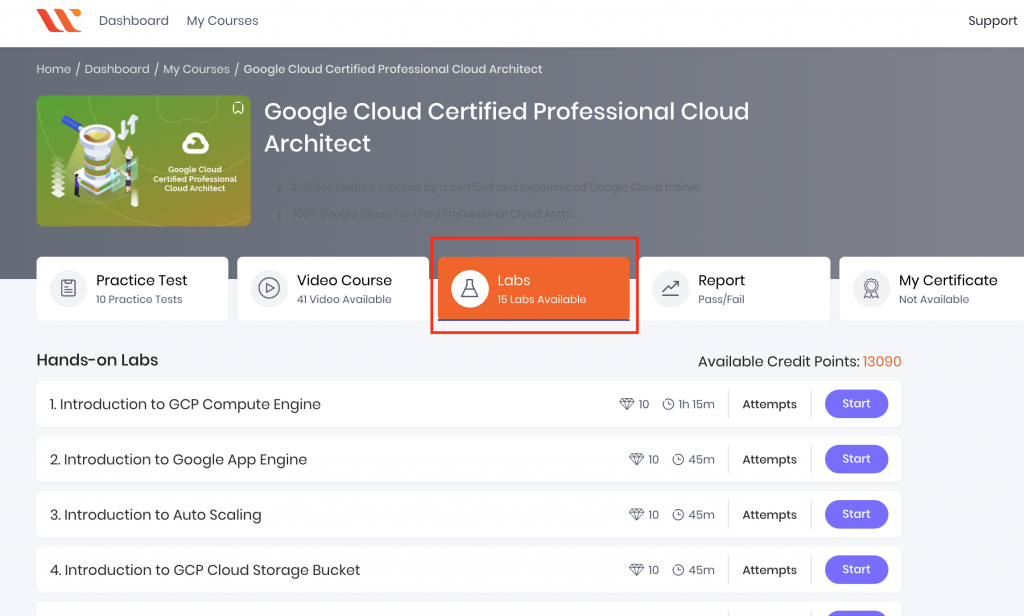The image is a screenshot from a computer displaying a website called Dashboard. The screen is segmented into various sections, each offering a specific functionality or information to the user. 

At the top, there is a navigation bar with tabs labeled Home, Dashboard, My Courses, and Google Cloud Certified Professional Cloud Architect. Below this bar, a portion of the screen prominently features the Google Cloud Certified Professional Cloud Architect, accompanied by an image representing this certification. This section is set against a green background and includes text that reads "Google Cloud Certified Professional Cloud Architect" with details such as "Practice Test," "Video Course," and "Labs" highlighted in red. 

A user has emphasized this section by drawing a red rectangle around it. Adjacent to this highlighted area, there is a section labeled "Reports" that features pass-fail statistics. Further down, there is a section titled "My Certificate," which displays the status as "Not Available."

On the right side of the screen, additional features are listed, including "Hands-on Labs" and "Available Credit Points," with the latter's value displayed in red text. Blue "Start" buttons are also visible, presumably providing access to various courses or activities.